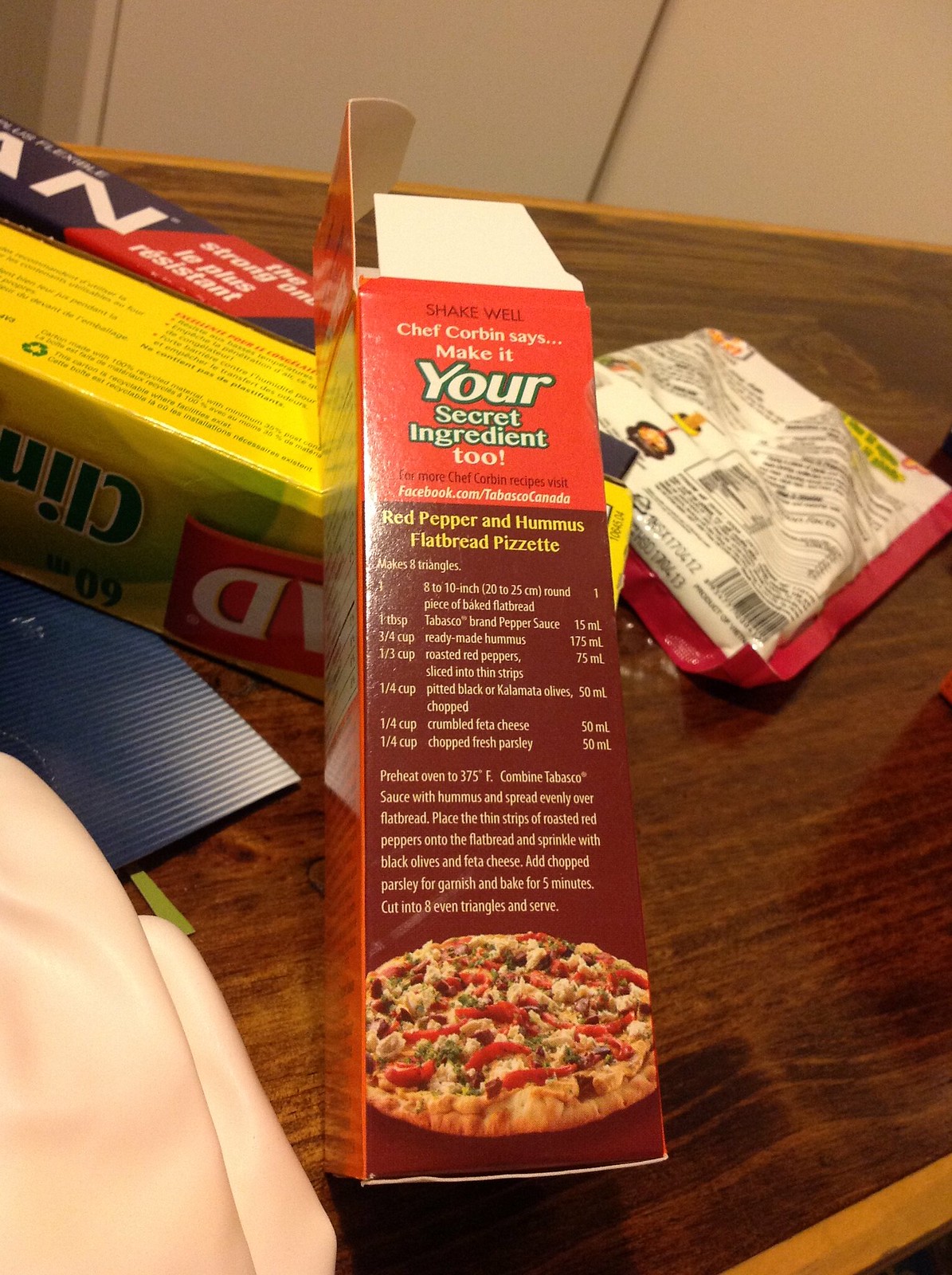The image showcases a cluttered wooden table featuring a vibrant red and maroon rectangular box prominently in the foreground. The box, which previously held a bottle of Tabasco sauce, is marked by informative text, including the line "Chef Corbin says, make it your secret ingredient too," and promotes additional recipes at "facebook.com/TabascoCanada." The box also presents a recipe for a red pepper and hummus flatbread pizzette, hinting at a fusion of Middle Eastern and Italian cuisine. An image of a supreme-style pizza with peppers and meat decorates the bottom of the box, complementing the recipe details. Surrounding this primary box on the table are various packaged goods: a distinguishable box of GLAD cling wrap and possibly a packet of taco seasoning with visible text, but too small to decipher. Adding to the assortment, there's potentially a box of aluminum foil marked “the strong one,” displayed in both English and French. All these items rest atop a finely grained wooden surface, with a white paneled wall in the background.